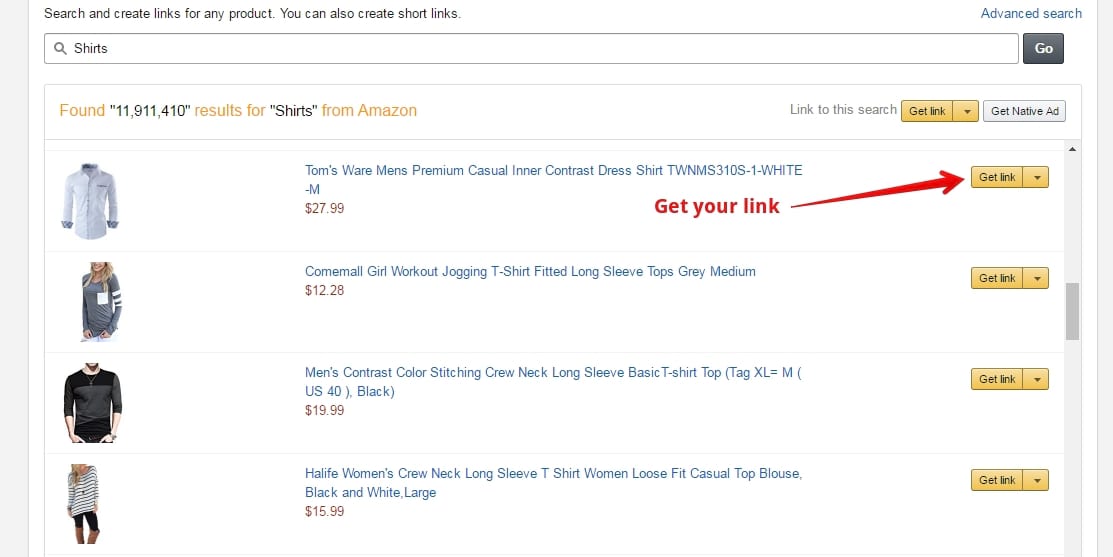This is a detailed screenshot from an Amazon website. At the top, a header states, "Search and create links for any product," with additional options to create short links and perform an advanced search. Below this header, a search bar with a magnifying glass icon on the left contains the query "shirts." The search has returned 11,911,410 results for shirts on Amazon.

On the left side of the interface, there are images of various shirt styles. The displayed items include:
1. A long-sleeved white shirt with gray rolled-up cuffs.
2. A fair-skinned blonde woman modeling a long-sleeved gray shirt with a white pocket on the right side and white horizontal stripes on the sleeves.
3. A man wearing a black and gray quarter-sleeve shirt.
4. A young fair-skinned blonde woman in a long white shirt with horizontal black stripes.

To the right of these images, the names and details of the items are listed:
1. "Tom's Wear Men's Premium Casual Inner Contrast Dress Shirt, TWNMS310S-1-WhiteM" priced at $27.99.
2. "COMEMALL Girl Workout Jogging T-Shirt Fitted Long Sleeves Tops Gray Medium" priced at $12.28.
3. "Men's Contrast Color Stitching Crew Neck Long Sleeve Basic T-Shirt Top Tag XL equals M US 40 Black."
4. "HALIFE Women's Crew Neck Long Sleeve T-Shirt Women's Loose Fit Casual Top Blouse Black and White Large."

A red arrow points to a yellow rectangle on the side of the screen that says "Get Link." Next to the arrow, in red letters, it reads "Get Your Link."